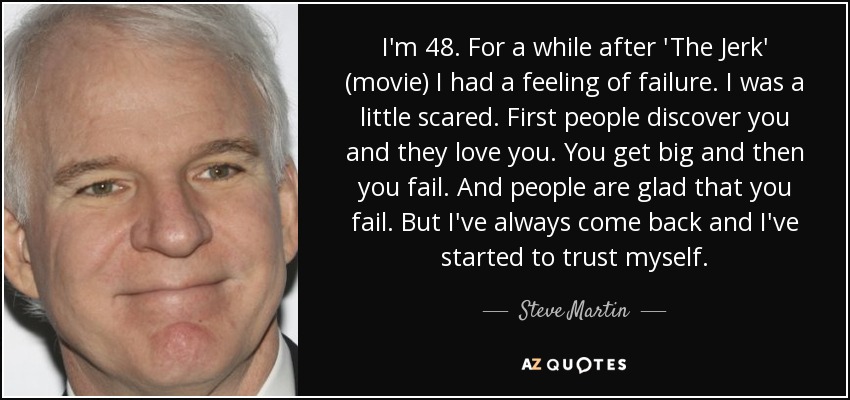This horizontally rectangular image features a full-color photograph of the actor and comedian Steve Martin, who is smiling with closed lips. His white or gray hair is clearly visible, and he is looking directly at the camera. Steve Martin, a white male, is dressed in a white collared shirt. The photograph is positioned in a small box on the left side of the image. The background has a black border, and the right side of the image contains a large black box with white text.

The text reads: "I am 48. For a while after The Jerk (movie), I had a feeling of failure. I was a little scared. First, people discover you and they love you. You get big, and then you fail. And people are glad that you fail. But I've always come back, and I've started to trust myself." 

Below the text is Steve Martin's autograph, followed by the words "AZ Quotes."

This image may be a screen capture, poster, or meme and is likely set indoors, given the photographic style.